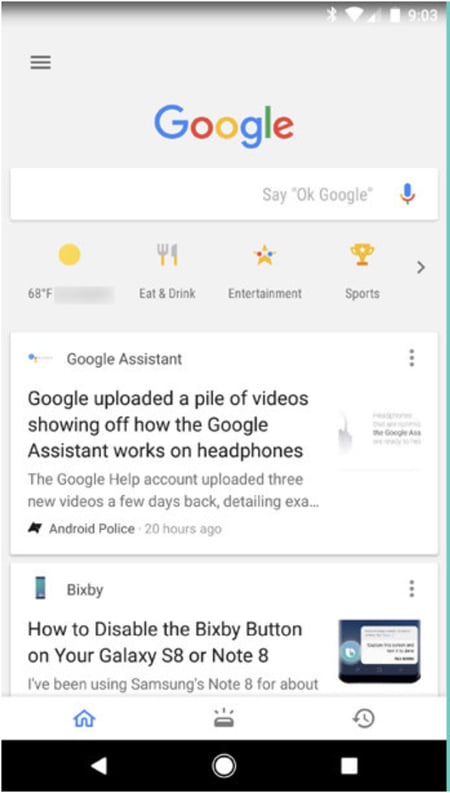This image is a screenshot taken from a smartphone displaying the Google home page. The time in the upper right-hand corner reads 9:03. The background of the page is a light gray. In the center, the iconic Google logo is prominently featured, with its vibrant blue 'G', red 'O', yellow 'O', blue 'G', green 'L', and red 'E'. Directly beneath the Google logo is the search box, a white oblong shape with the prompt "Say 'Ok Google'" to the right. Next to this prompt is a small microphone icon, indicating the option for voice search.

Below the search box, the temperature is displayed as 68 degrees Fahrenheit, though the city name appears to be blotted out. Adjacent to the weather information are quick-access categories labeled "Eat and Drink," "Entertainment," and "Sports."

Further down, there is a white rectangle labeled "Google Assistant." A description notes that "Google uploaded a pile of videos showing off how the Google Assistant works on headphones." Following this, another white box appears, labeled "Bixby," along with a guide titled "How to disable the Bixby button on your Galaxy S8 or Note 8."

At the very bottom of the screenshot, the footer is black with a white square to the right, an arrow on the left, and a white circle in the center.